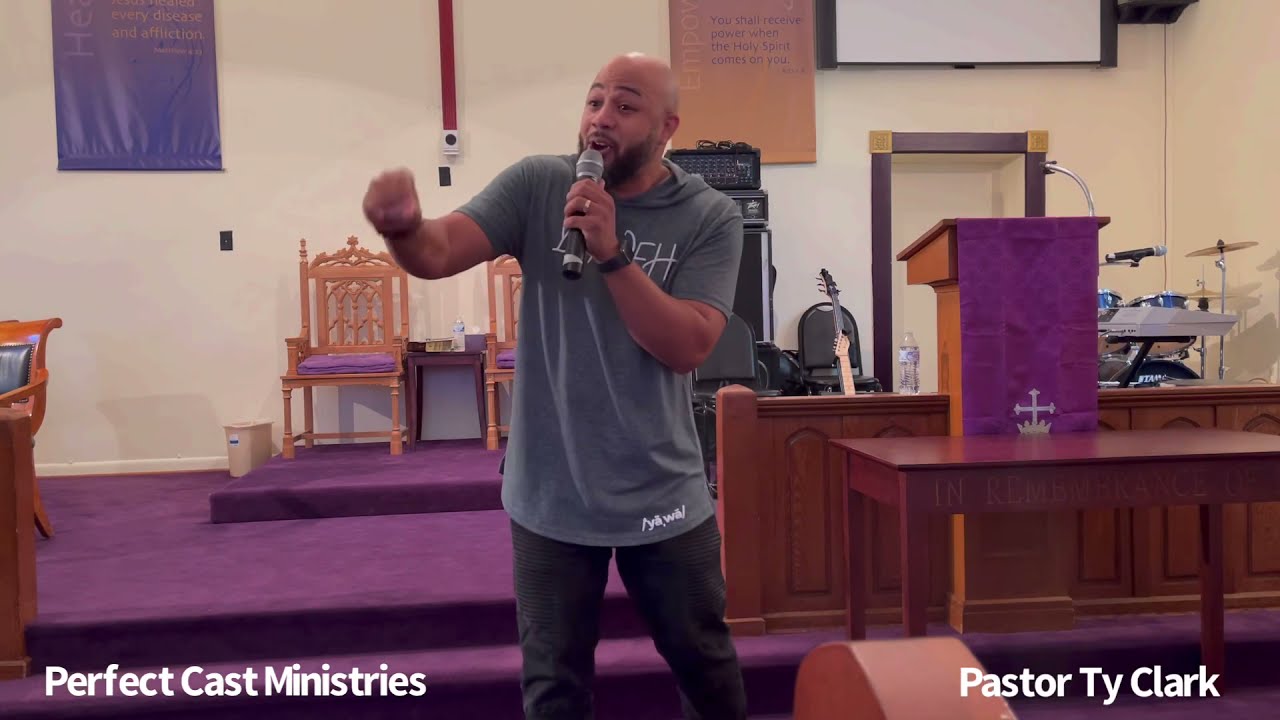In the image, a man identified as Pastor Ty Clark is seen dynamically addressing an unseen audience. He is wearing a gray, short-sleeved t-shirt with a hood, black pants, and a wedding ring. His left hand grasps a microphone, while his right hand, clenched into a fist, points forward as he speaks. The scene is set inside a beige-walled building, with a podium draped in a purple cloth adorned with a cross positioned to his right. In front of the podium, a wooden table inscribed with "In Remembrance" stands prominently. The platform area behind him is carpeted in purple, and features a musical setup with a drum set, a guitar, and speakers. Two wooden chairs with purple cushions are placed on a slightly elevated section, separated by a wooden railing from the pastor's area, which is two steps below. Additional details include a white projection screen and various posters on the wall. The lower corners of the image display text in white font reading "Perfect Cast Ministries" on the left and "Pastor Ty Clark" on the right.